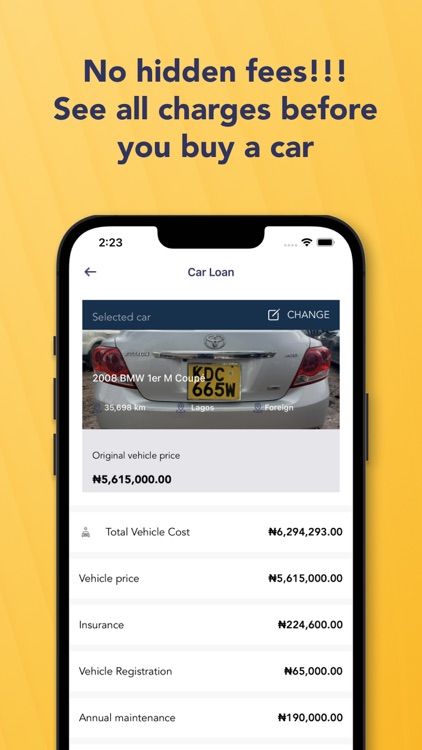This graphic features a rectangular layout with a vibrant background transitioning from shades of light yellow to dark yellow, bordering on orange, and darkening further towards the lower right corner. This gradient effect evokes the warmth and radiance of sun rays.

Centered at the upper portion of the graphic, bold black text commands attention with the phrase "NO HIDDEN FEES!!!" followed by the statement, "See all charges before you buy a car."

Beneath this text, a prominent image of an illuminated smartphone displays a website related to car loans. The screen details various costs associated with purchasing a vehicle, including total vehicle cost, vehicle price, insurance, registration, and annual maintenance, all in black font against a white background.

Central on the smartphone's screen is a rectangular picture of a car viewed from the rear. The car is depicted in white or possibly a light gray/silver color, featuring a square yellow license plate inscribed with "KDC665W". 

The detailed information presented across the graphic underscores the emphasis on transparency in car purchasing, reinforcing the message of no hidden fees.